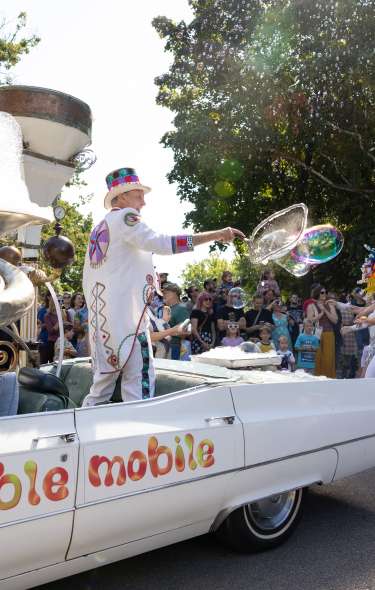The image captures a vibrant parade scene, focusing on an older white Cadillac convertible, primarily viewed from the rear angle, featuring a distinctive back wheel. A man, exuberantly standing in the back seat, commands attention. He's dressed completely in white, with a noticeable top hat and detailed designs in cyan, purple, and red on his long jacket. He joyfully wields a giant bubble wand, creating a mesmerizing cascade of bubbles using soapy material from a pan. The side of the convertible displays the partially obscured word "mobile" in bold red letters. Surrounding him, a crowd of families and children gleefully watch, some applauding, fully engaged in the spectacle. The setting is adorned with lush, leafy green trees, particularly a large deciduous one in the upper right corner, amidst a backdrop of a white sky, hinting at an overcast day. A conspicuous yellow cone on the left adds a peculiar touch to the scene, amidst the ambient excitement of the parade. The sunlight softly illuminates the bubbles, casting iridescent hues that enhance the festive atmosphere.